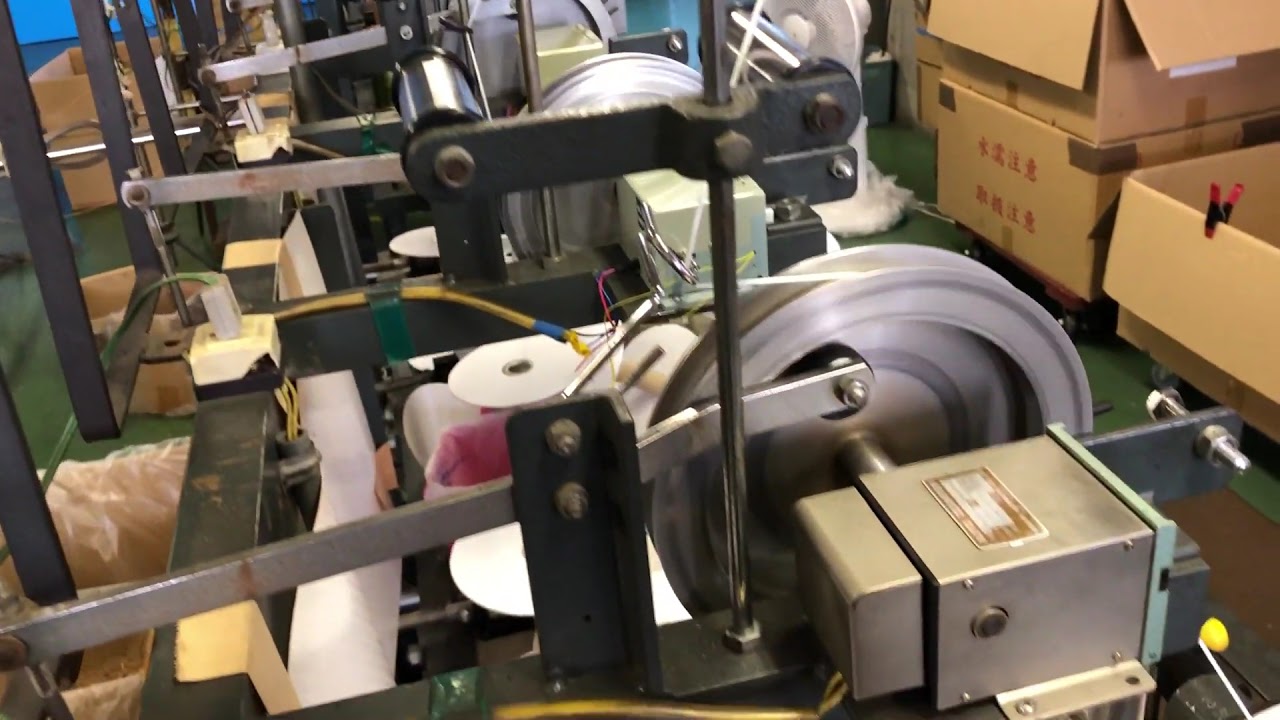The image depicts an indoor workshop or factory setting characterized by rows of machinery and various engineering components. Centrally positioned, the machinery includes several large, metal spinning wheels, one of which features a yellow and white string or wire attached. The workshop appears cluttered with exposed wiring, pipes, and metal bars held together by numerous screws, showcasing a variety of tools and components in organized rows of shelving. On the right side of the image, there are several boxes with plastic linings, some of which contain non-English, possibly Chinese, text. The upper right corner houses more boxes stacked together. The setting is further defined by a green epoxy floor, adding to the industrial ambiance. This detailed scene suggests ongoing production and packaging activities, though the specific items being manufactured or their purposes remain unclear.